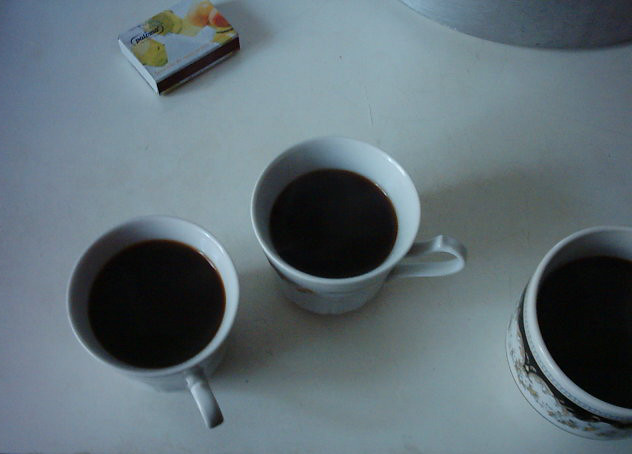The photo captures a white tabletop scene with a light source casting shadows from three containers onto the surface. Dominantly, there are three vessels each containing a dark liquid, presumably coffee. Two are white, identical mugs placed on the left and center, while the third, positioned at the bottom right, is larger, rounder, and adorned with a black and tan pattern. In the upper left corner, there is a matchbook decorated with orange, yellow, and possibly peach fruit designs. Additionally, an unidentifiable gray object is situated in the upper right corner, adding a touch of mystery to the arrangement.